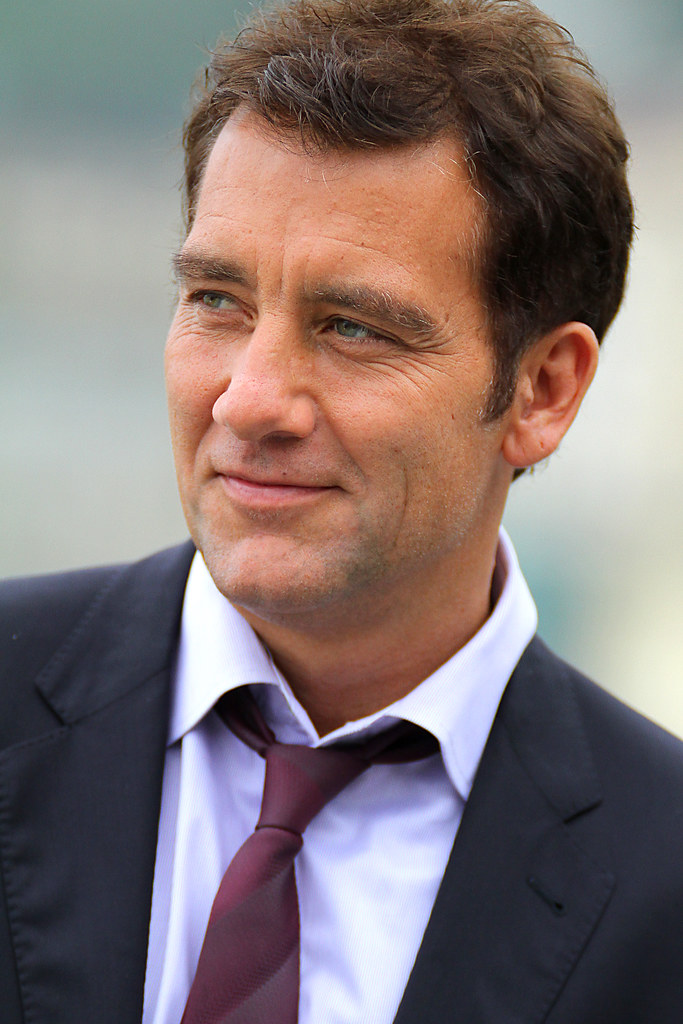In this detailed photograph, a man occupies the center of the frame, gazing slightly off to the left with a subtle, closed-mouth smile. His greenish-blue eyes, framed by light wrinkles, suggest a slight squint as he looks off into the distance. The man sports a neatly trimmed stubble of mixed brown and gray on his cheeks and upper lip, complementing his dark brown hair, which is slightly messy and brushed to the left, showing a few strands of gray.

He is dressed formally in a dark-colored business coat, possibly black or dark blue, paired with a crisp white button-up shirt, the top button left undone for a more relaxed look. Around his neck, he wears a distinct red and gray striped tie, the colors adding a touch of contrast to his outfit. One of his ears is visible, showing holes indicative of past piercings.

The background, though out of focus, hints at an outdoor setting and does not distract from the subject. The man's shoulders are slightly angled, enhancing the natural, candid feel of the photograph, which is likely taken in daylight. The overall color palette features black, white, and various shades of red, contributing to the refined yet approachable impression conveyed by the image.